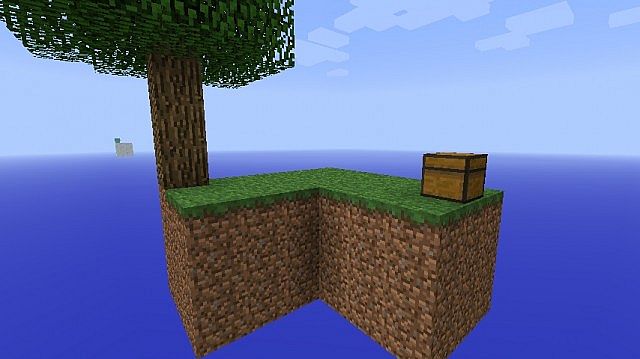This image depicts a scene from the popular video game Minecraft, developed by Mojang. The landscape features the game's characteristic blocky texture and simplistic graphics. At the center of the image is an L-shaped floating island. A large tree, comprising brown blocks simulating the trunk and green blocks for the foliage, dominates the island's narrow surface. 

Attached to the green canopy of the tree is a brown chest with black trim, blending seamlessly into the lush green grass that covers most of the island's top surface. Below the grassy platform, the island's base consists of blocks resembling dirt, which further reinforces the floating illusion commonly seen in Minecraft environments.